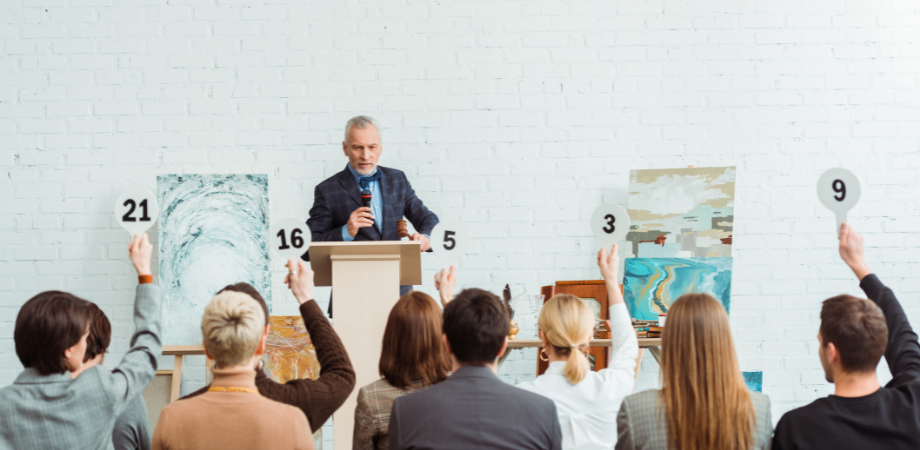In the detailed photograph set inside an art gallery, a lively auction is taking place against the backdrop of a white brick wall. At the podium stands an auctioneer, distinguished by his dark blue-gray pinstripe suit, light blue button-up shirt, and blue bow tie, holding a gavel in his right hand and a black and red microphone in his left. He has gray hair, a gray goatee, and mustache. Flanking him are two paintings on easels: the one to the left is predominantly blue and white, while the one on the right depicts a serene scene with clouds and sea in shades of brown, light blue, and dark blue. Additional artworks, including clay objects, are displayed against the wall and on a table. In the foreground, nine attendees seated in chairs actively participate, holding bidding paddles with numbers 3, 5, 9, 16, and 21. The man holding paddle number 9, positioned in the bottom right corner, wears a long black shirt and has brown hair.